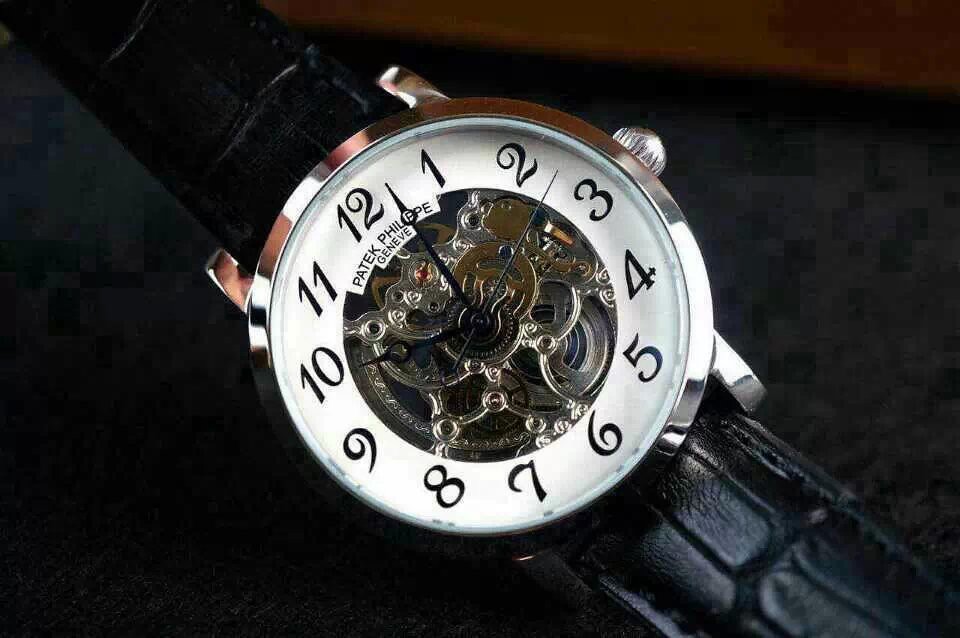This image features a luxurious and sophisticated Patek Philippe watch. The timepiece boasts a white face with a meticulously crafted cutout center, offering a glimpse of the intricate gears beneath—a testament to its high-end craftsmanship. The Arabic numerals, elegantly rendered in cursive, display the hours from 1 through 12. Prominently positioned just below the 12 o'clock marker, the watch face is adorned with the prestigious branding "Patek Philippe" followed by "Geneva." The watch is further equipped with an hour, minute, and second hand, completing its classic yet exquisite design.